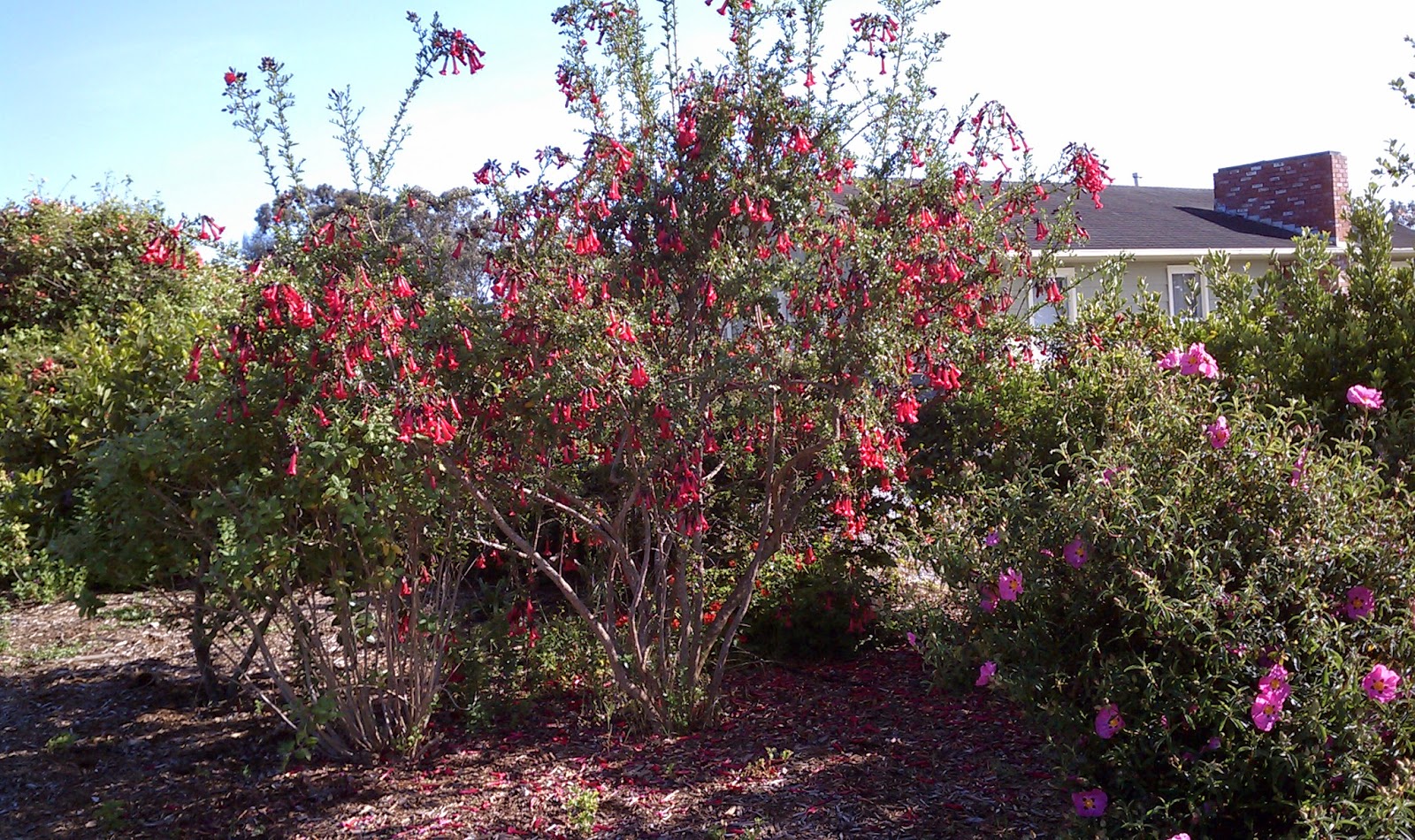This vibrant photograph showcases a lush backyard garden densely populated with various plants and flowers, which partially obstruct a small, single-level home in the background. The house, featuring a brown roof and a distinct diagonal brick chimney on the right, peeks through the rich greenery. Dominating the scene are two prominent taller trees or bush-like plants in the center, adorned with red flowers that appear to be either budding or withering. To the right, a bush boasts striking pinkish-purple blooms, which add a pop of color. The left side reveals more trees and plants against the backdrop of a clear blue sky. Grounded in a layer of mulch or sand, the garden also includes multiple green bushes that, though flowerless, contribute to the verdant, serene atmosphere of the photo.